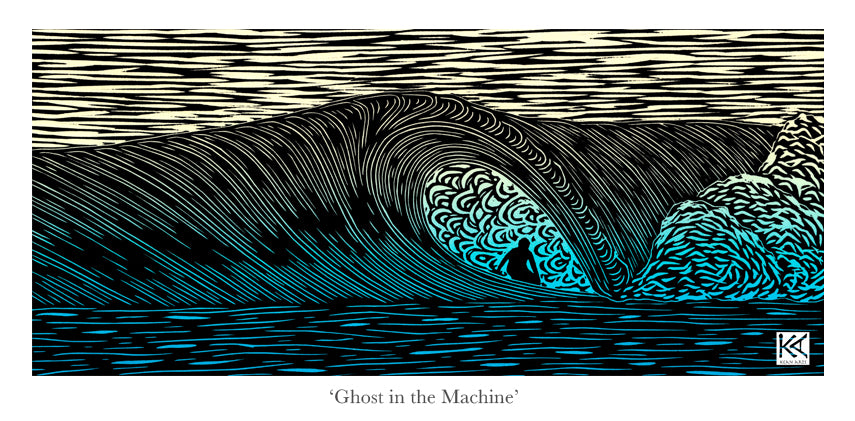This captivating hand-drawn painting, titled "Ghost in the Machine," features a dramatic depiction of a surfer riding the curl of a massive wave. The wave itself is presented in a striking combination of deep black, bright blue, and various vibrant hues, accentuated with intricate white and blue stripes indicating the water's momentum and foam. The upper section of the image showcases a woven-like pattern of black and white, representing the sky. The central focus of the painting is the surfer, situated in the bright blue center of the curling wave, masterfully highlighted by black sweeping lines that suggest both the motion and power of the water. Additional abstract elements in turquoise, orange, and aqua tones add depth and dynamism to the scene, enhancing the visual complexity. At the base of the wave and on the right side, the artist employs black and blue strokes to portray the water's reflection and foam. The image boasts a wide horizontal format with heavy use of black ink and vivid colors, emphasizing its bold graphic style. In the bottom right corner, a watermark bearing the initials "K.A." is visible, while beneath the drawing, the title "Ghost in the Machine" is printed in black Times New Roman font on a white background.